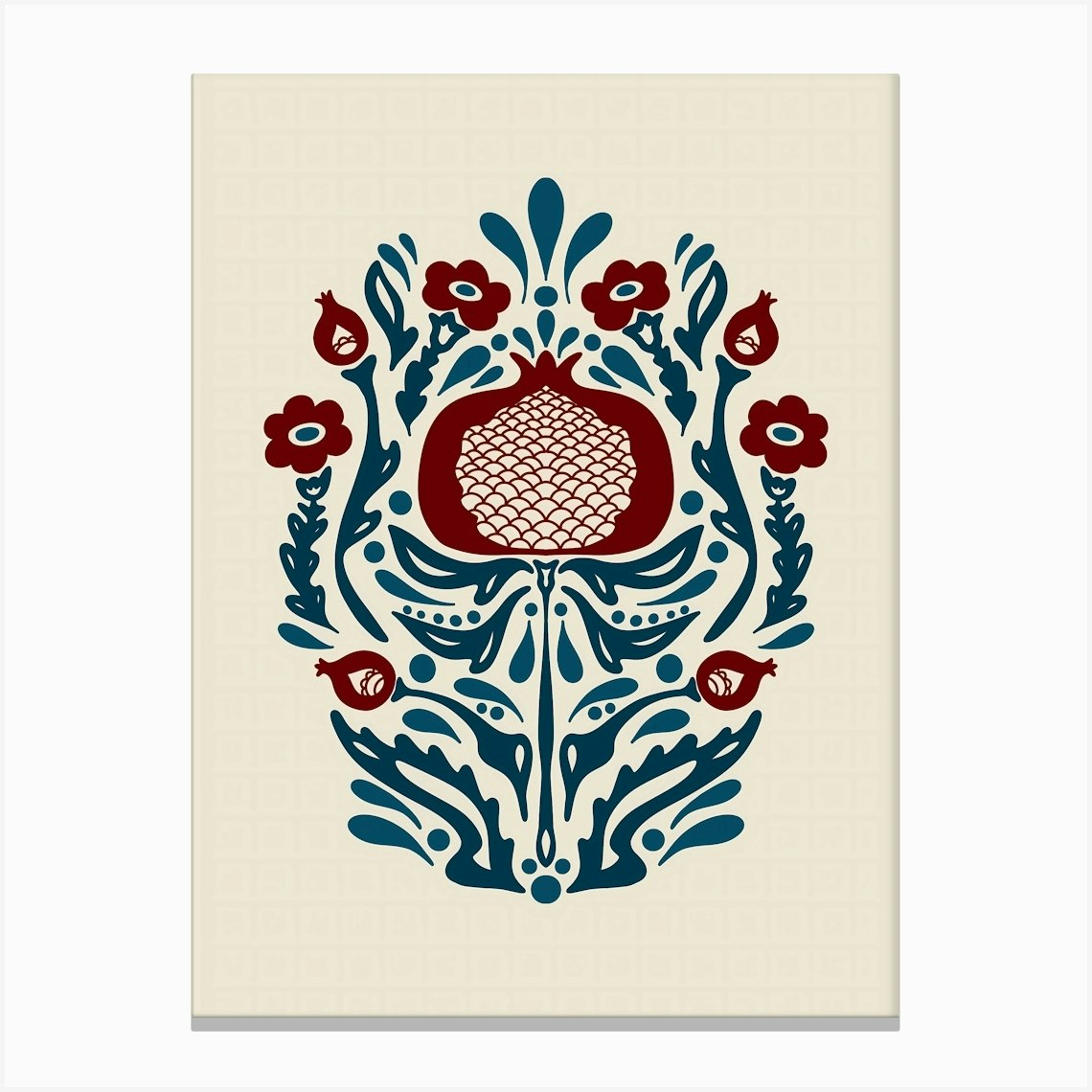This image depicts a highly stylized painting on a vertical canvas, framed against a solid white background. The canvas itself is of a cream color and features a composition dominated by dark greens and reddish-brown or maroon hues. The painting appears almost Rorschach-like in its symmetry and abstraction, giving it an enigmatic quality.

At the top center of the canvas, there is a large, reddish-brown bulbous structure that seems to resemble flowers or buds, intricately detailed with what looks like seeds in the middle. Surrounding this central element are symmetrical designs of leaves and stems rendered in dark green, adding to the floral motif of the piece.

The subtle, light, square patterns scattered across the canvas go mostly unnoticed unless scrutinized closely, as they do not interfere with the dominant figures of the painting. The overall effect is that of a detailed and symmetrical floral scene, meticulously crafted using a limited but rich color palette of maroon and green.